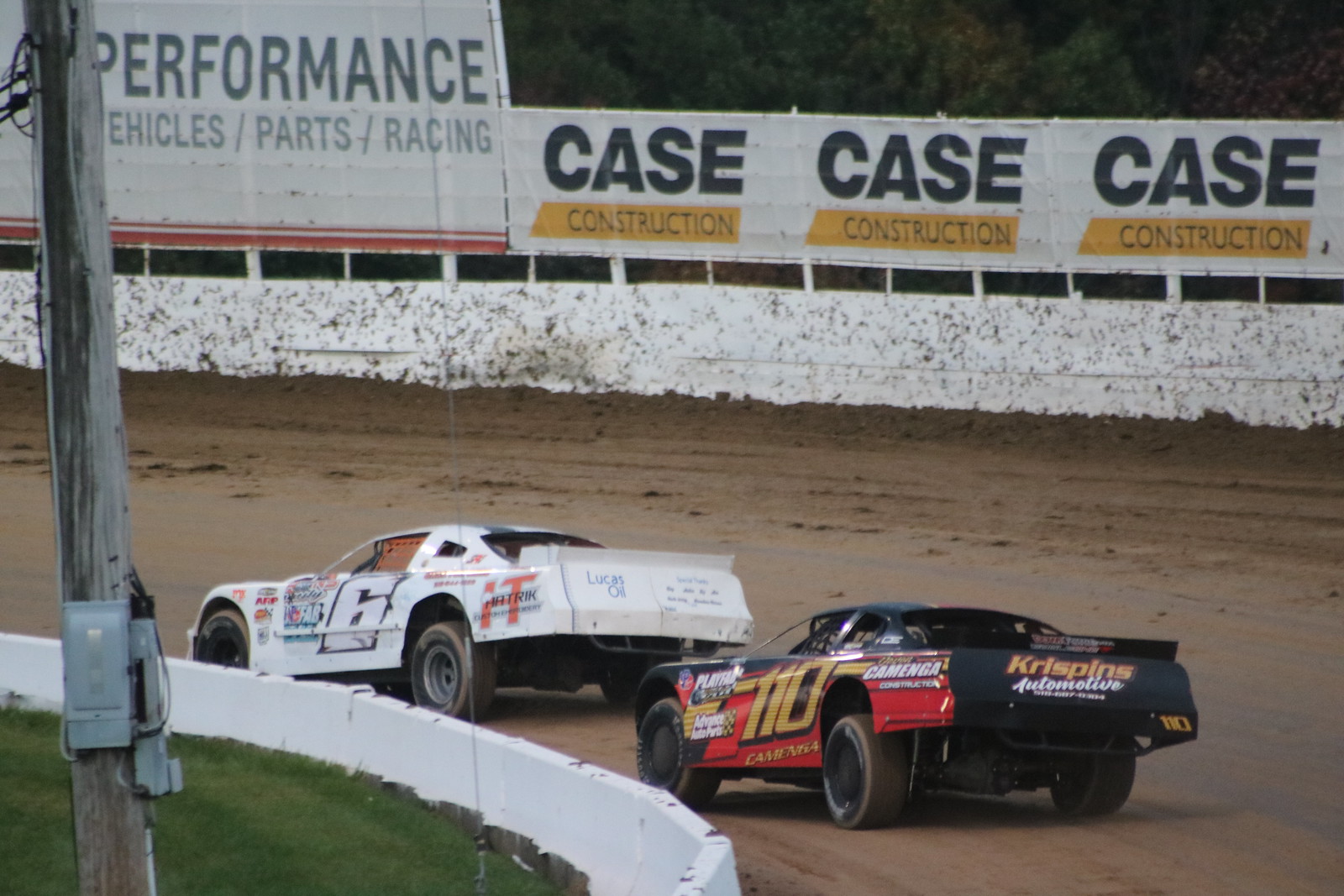The image captures an intense moment on a muddy, circular dirt track where two race cars are speeding around a curve. The scene is zoomed in to show part of the track and its surroundings in vivid detail. The track, composed entirely of dirt and looking particularly muddy, is bordered by a splattered white barricade wall. Advertisements are prominently displayed on this wall, including those for Case Construction and Performance Vehicle Parts Racing. The inner side of the track features a white barrier that separates the dirt surface from a green grass area at the center. Within this grassy area is a tall, wooden utility pole equipped with metal boxes at its base.

Leading the race is the white number 6 car, which has multiple advertisements including one for Lucas Oil. Behind it is the black number 110 car, distinguished by red decorations on its side panel, an orange banner for Crispin's Automotive, and a yellow number. Both cars appear to be moving at high speed, adding a dynamic sense of motion to the photograph.